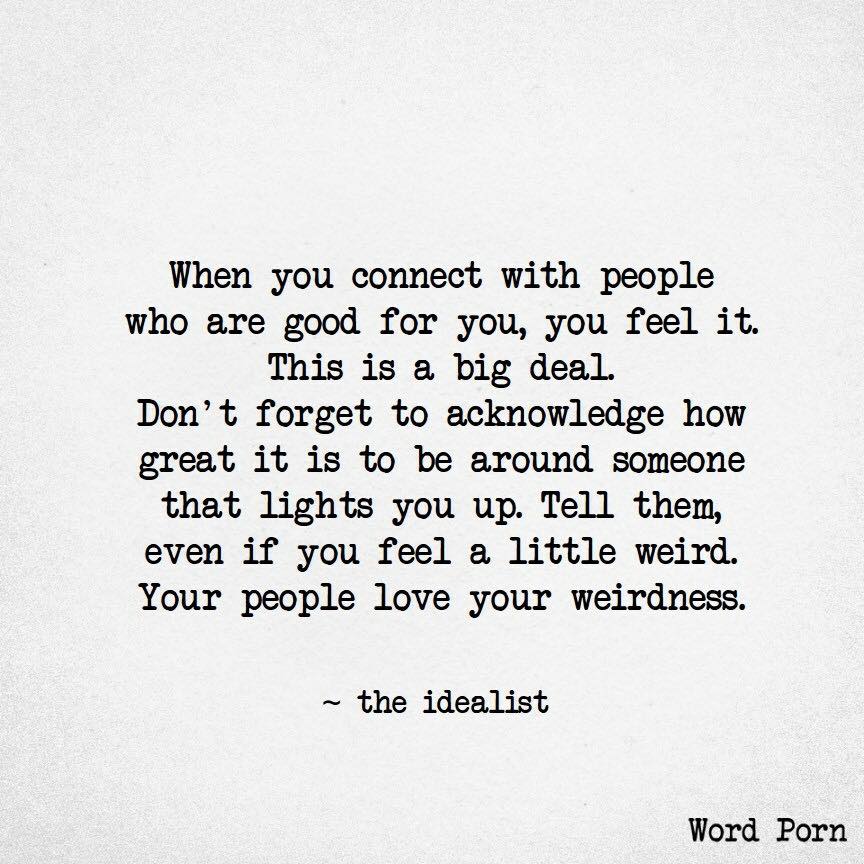This text-based image, with an off-white background that has a textured gray pattern, features a motivational message in black, typewriter-style font. The centered text reads: “When you connect with people who are good for you, you feel it. This is a big deal. Don't forget to acknowledge how great it is to be around someone that lights you up. Tell them, even if you feel a little weird. Your people love your weirdness.” Below the main text, a tilde is followed by “the idealist” in lowercase letters. The bottom right corner of the square image is signed “WordPorn” with capital W and P.